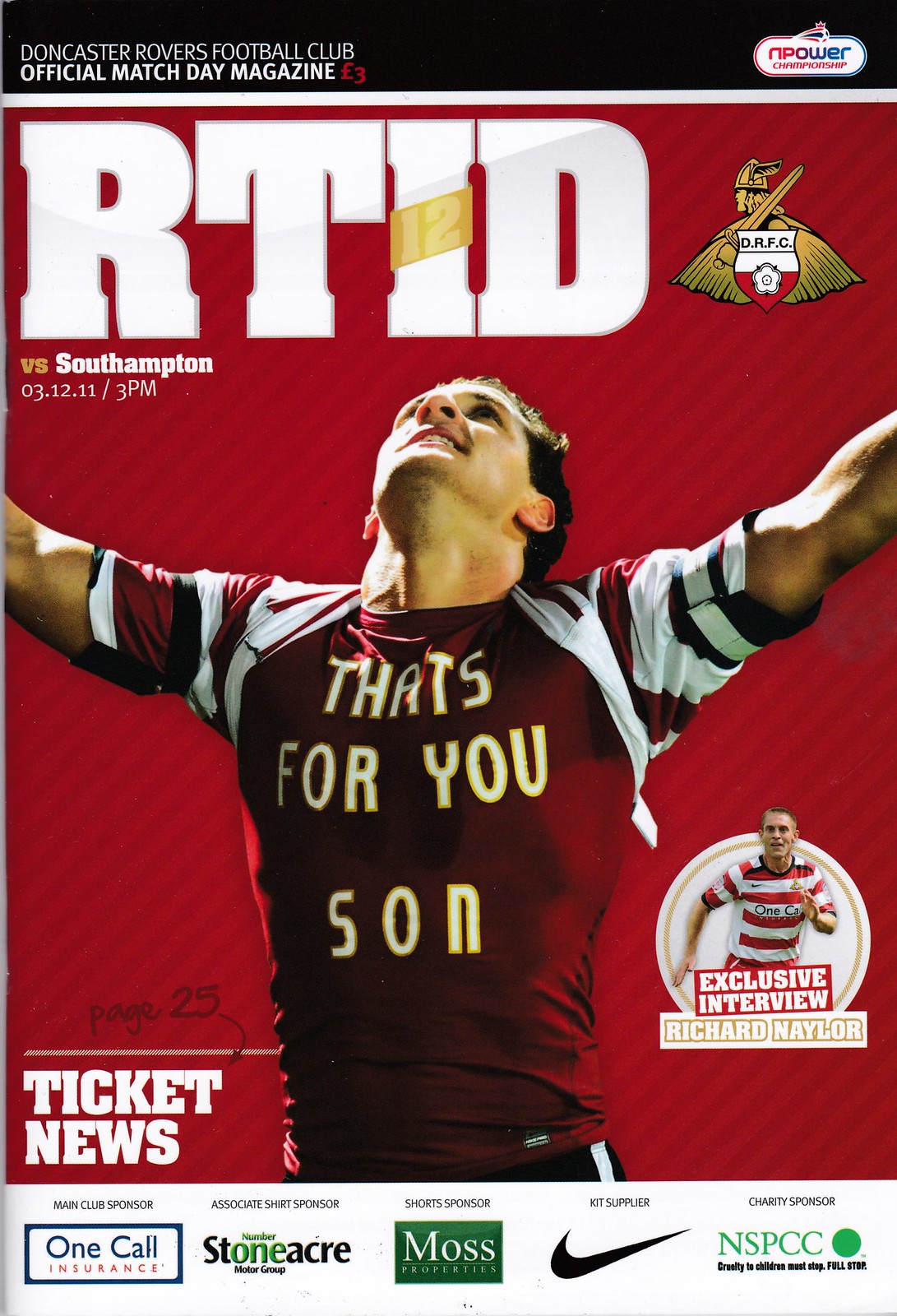The front cover of the Doncaster Rovers Football Club Official Match Day magazine is prominently red with a detailed layout. At the very top, a black strip reads "Doncaster Rovers Football Club Official Match Day Magazine" in white text, and "three pounds" in red. In the upper right corner, the logo "NPower Championship" is displayed, with 'NP' in red and 'ower' in blue. Below, large white letters spell out "RTID" with a yellow strip wrapped around the letter "I" that says "12" in light gray. The game details "vs. Southampton" and "03.12.11 3 p.m." are listed underneath.

The main image features a football player with outstretched arms, wearing a red short-sleeve shirt with white stripes on the sleeves. The player's jersey is emblazoned with "That's for you son". There's also a smaller image of another person in a shirt with horizontal red and white stripes, and a sticker/banner announcing an exclusive interview with Richard Naylor. Additional information includes ticket news on page 25. At the bottom of the cover, various sponsors are listed: Stoneacre, Moss, Nike, One Call Insurance, and NSPCC. The overall design conveys excitement and anticipation for the upcoming match.